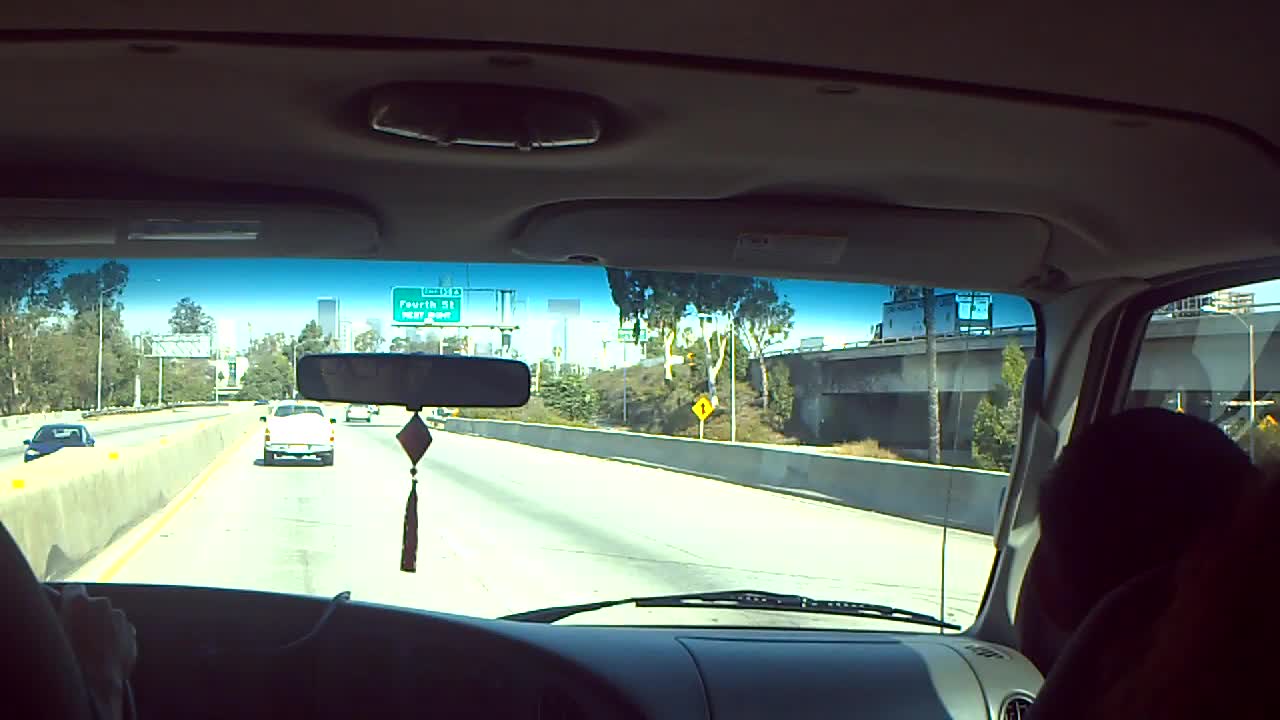The photograph captures a scene from inside a car, taken through the front windshield, most likely from the back seat. The silhouettes of two people are visible: one on the right, seated in the front passenger seat, and the other on the left, their hand on the steering wheel, indicating they are the driver. The lack of interior lighting contrasts with the bright conditions outside, overexposing the road. 

Through the windshield, the vehicle is traveling on a highway, passing an exit that might be marked 135A or 153A, leading to 4th Street. The exit sign indicates it will be on the next right. A light-colored truck is directly ahead, with two other cars traveling in the same direction. On the opposite side of the highway, separated by a cement divider, a darker car is visible traveling in the opposite direction. 

The weather is notably bright, and the sky is clear blue. In the distance, a city skyline with tall buildings can be seen, framed by trees lining both sides of the highway. Inside the car, a decorative tassel with a diamond-shaped pendant hangs from the rearview mirror, adding a personal touch to the otherwise typical vehicle interior.